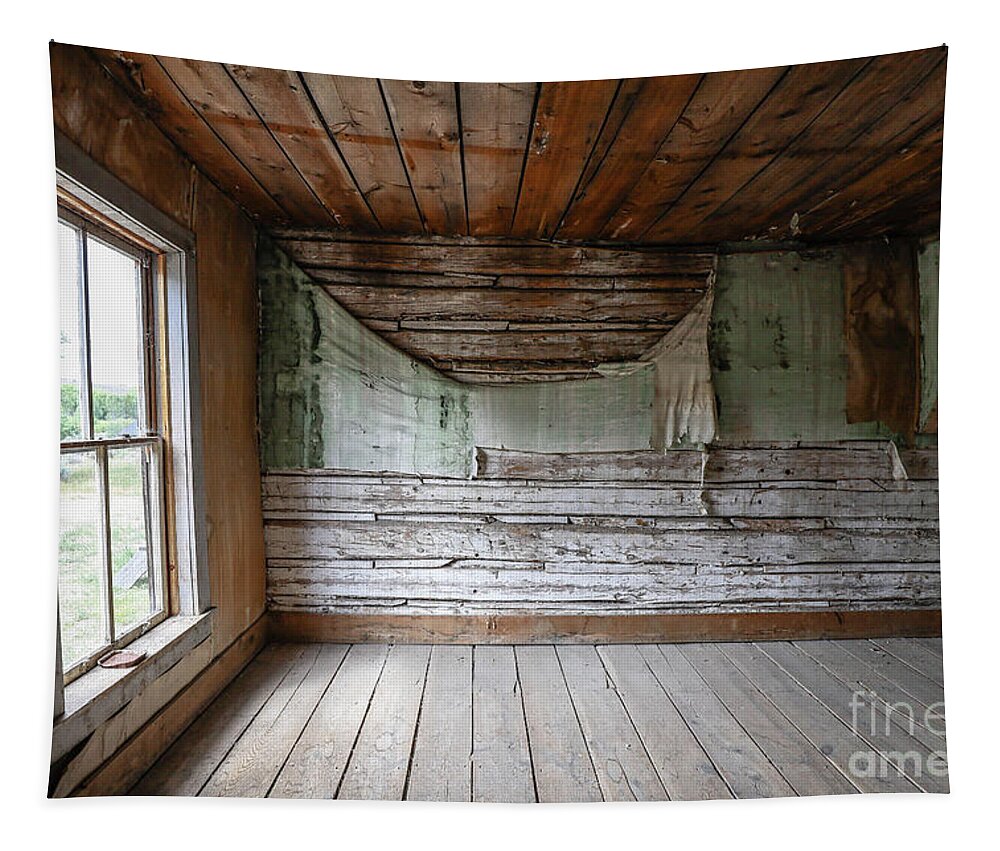The image depicts the interior of an old, possibly abandoned wooden cabin. The room is bare and unfurnished, with aged, dusty wooden planks making up the floor and walls. The walls, which are cracked and weathered, feature a large four-pane window that allows a view of a faintly visible green exterior, suggestive of a beach environment rather than a mountainous one. Details outside the window are sparse, with only a few bushes and some grass discernible. Dominating the scene, the wooden ceiling appears to be bowed under weight, reinforcing the cabin's dilapidated state. A fabric, likely a rug once hung for warmth, now hangs listlessly from the main wall, tattered and partially fallen. The ceiling planks are notably a deeper, richer brown compared to the rest of the wood. There's also a watermark in the image that reads "fine AME," though it’s incomplete and unclear what it fully denotes. The cabin evokes a strong sense of antiquity and abandonment, highlighted by its faded, unfinished appearance and the overall decrepitude of its interior.